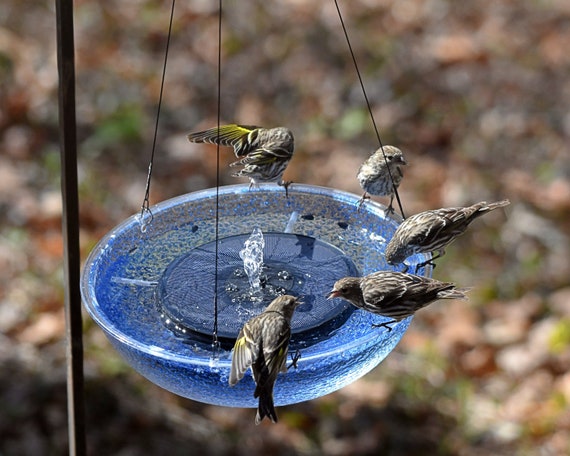This engaging wildlife photograph captures five lively birds perched around the edge of a hanging, round birdbath. The birdbath is a crystal-clear bowl with a slight blue tinge and a textured, pebbly appearance, suspended by three cords attached to loops at its edges. At its center, a device causes water to bubble and spurt up a few inches, providing a playful element for the birds. Some birds appear to be drinking the bubbling water, while others are interacting as if chatting and surveying their surroundings. Notably, one bird is delightfully bathing in the refreshing water. The background, though blurred, seems to suggest a leafy forest floor, with earthy browns dominating the scene. The birdbath is hung from a pole, contributing an element of charm to this picturesque, serene outdoor setting.